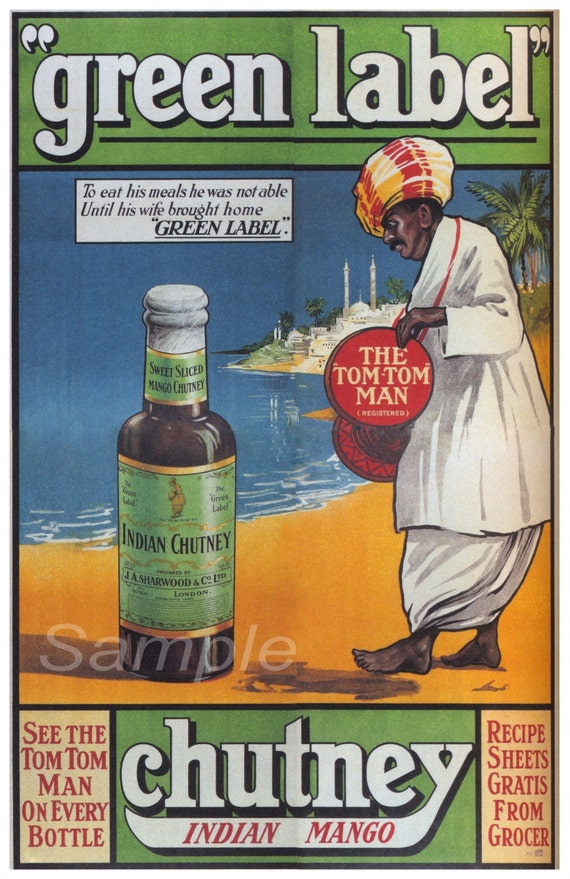This full-page advertisement, likely from the 1950s or 60s, is aesthetically illustrative and vividly captures an exotic beach setting. At the top, a green rectangular header spans the width of the page, with bold white text outlined in black that reads "green label" in quotations. Below this header, the main illustration dominates two-thirds of the page, featuring a darker-skinned Indian man standing barefoot on yellow sand, in front of a serene blue ocean with green palm trees and a white building reminiscent of the Taj Mahal in the background.

The man, adorned in a yellow and red turban and wearing a white long shirt with poufy, tapered white pants, holds a red circular sign that says "Tom Tom Man" in yellow text. A significant feature of the ad is the large brown bottle with a white cap, situated prominently in front of the man, bearing a green label that reads "Indian chutney." Additionally, near the bottom of the bottle, the label specifies "chutney, Indian mango."

Supplementing the vivid visual are two red-text sections on either side at the bottom of the illustration. The left section reads, "See the Tom Tom Man on Every Bottle," while the right section proclaims, "Recipe Sheets Gratis from Grocer." This detailed and nostalgic advertisement encapsulates the cultural and commercial appeal of the product it promotes.